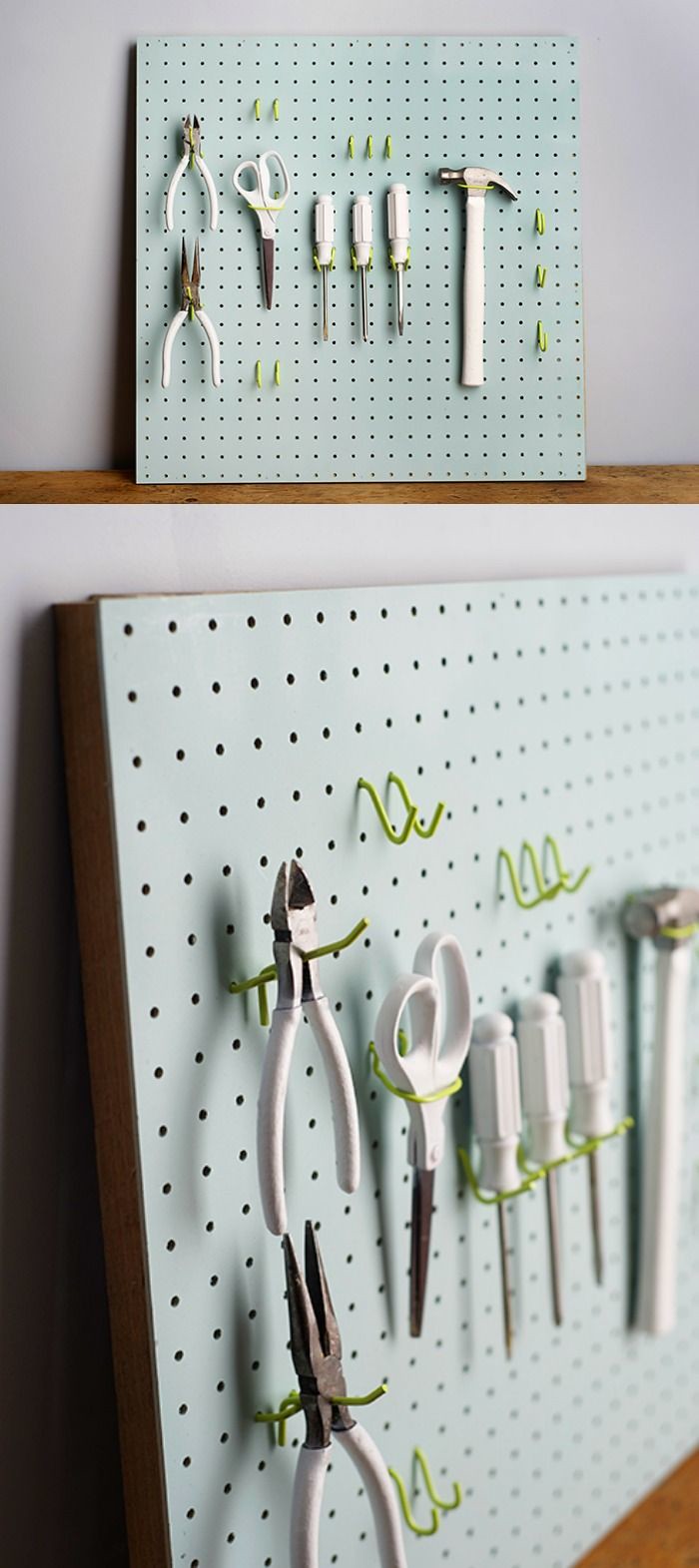This composite image features two photographs of an organized, blue pegboard commonly found in crafting or hardware settings, displaying an array of perfectly arranged tools. The collage consists of one wide, full shot of the pegboard and a closer, angled shot highlighting the area with pliers and a hammer. Both images capture identical pegboards, neatly mounted on a white wall with brown wooden molding at the top.

The pegboard itself has an array of lime green hooks, some of which are currently unused. The selection of tools, all featuring white handles, includes two sets of pliers—one needle-nose and one wire-cutter—next to a pair of scissors. Adjacent to them are three screwdrivers lined up in a row, followed by a hammer positioned at the end. The tools’ metallic parts gleam in the light, enhancing their clean, polished look.

In the close-up image, taken from the side of the pegboard showing the pliers, the white-handled hammer is just visible at the edge of the frame. The hooks and pegboard slots are intricately detailed, suggesting an eye-catching display, possibly staged for aesthetic purposes or efficient tool storage. The overall impression is one of organized efficiency, with a touch of visual appeal that makes the functional arrangement striking.